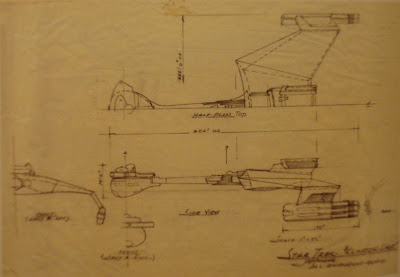This image showcases an aged, hand-drawn mechanical draft of a science fiction spacecraft from the Star Trek series, specifically resembling a Klingon warship, a known adversary of the USS Enterprise. Drawn on brown paper, which adds a vintage touch, the draft details the height, width, and shape of the vessel through multiple perspectives: a side view illustrating the control cockpit and main body with rocket engines beneath, a top view, and an angled view of the wing. Black ink sketches and various measurements are scattered across the paper, with the notable inclusion of a signature line labeled "Star Trek" in the bottom right corner, further cementing its origin in the iconic 1960s TV series.